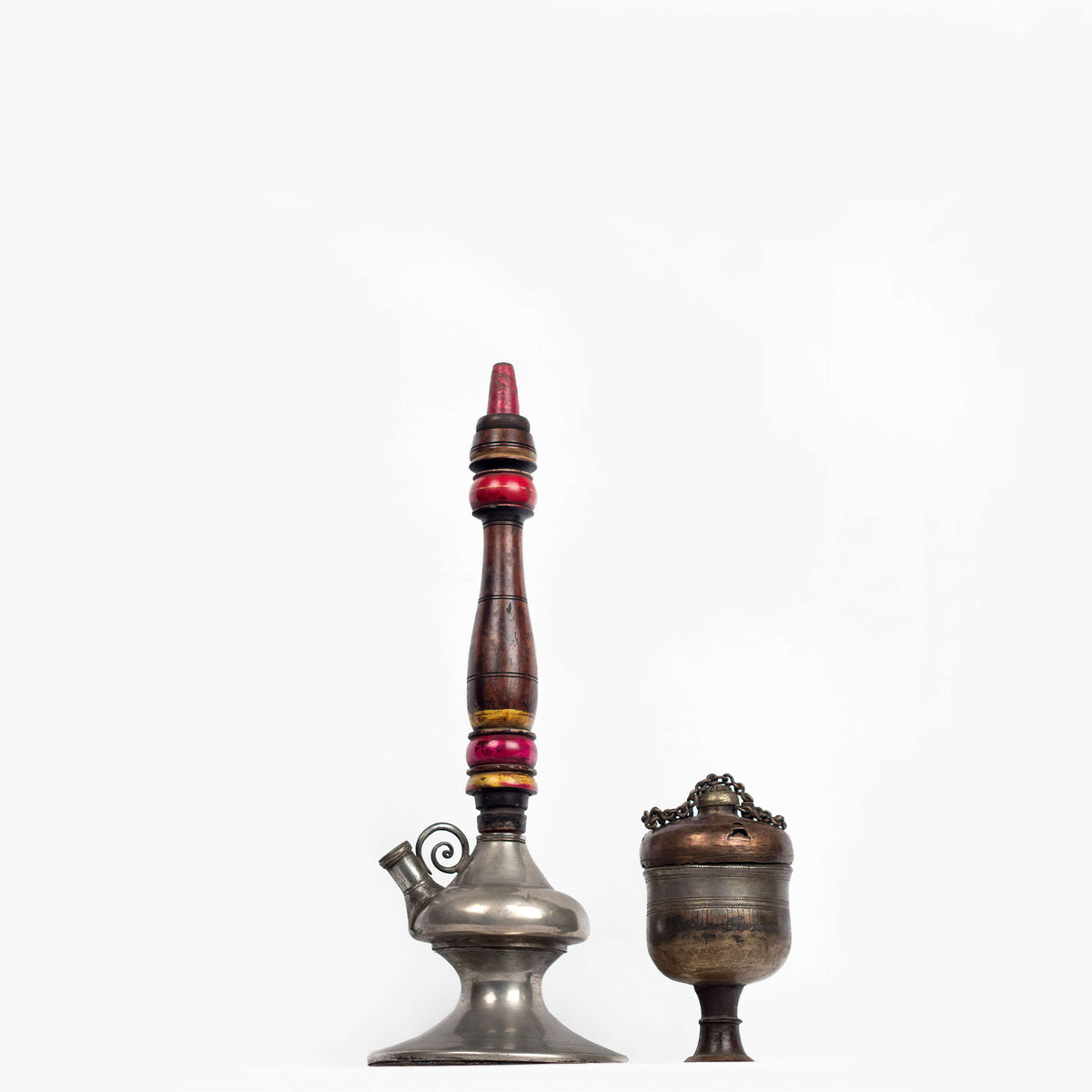This image showcases a detailed close-up of an ornate hookah pipe set against a white background. The base of the hookah is designed like a polished silver or chrome urn, reminiscent of a genie lamp, featuring a carved attachment point for the hose. Rising from the base is a tall, ornate tower-like structure made of turned wood, adorned with intricate brown and red patterns. Adjacent to the hookah is a smaller, rounded square container, possibly made of pewter or tarnished silver, and equipped with a chain on its lid, suggesting it might be used for storing tobacco or could be a religious chalice. The overall composition and elaborate design elements hint at a Middle Eastern influence.